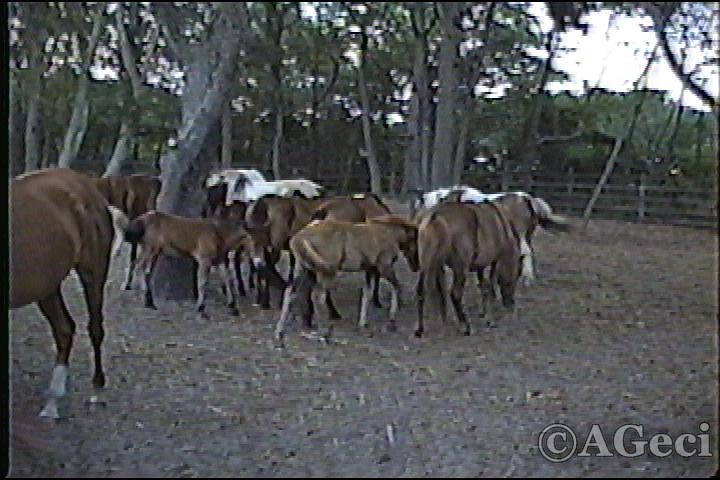The grainy, blurry image shows an enclosure filled with at least a dozen horses of various shades ranging from deep reddish-brown to golden-brown, with two or three white horses also present. They are mostly clustered together in the center of the frame, walking on a mix of dirt and wood chips. Among them are adult horses as well as foals, identifiable by their smaller size and thinner faces. The enclosure is surrounded by a wooden fence made up of horizontal beams fastened to vertical posts spaced two to three meters apart. In the background, a mix of brownish tree trunks and green leaves is visible, both inside and outside the enclosure. A possible structure appears faintly behind the trees. The image carries a watermark at the bottom that says, "Copyright A. Gechi."